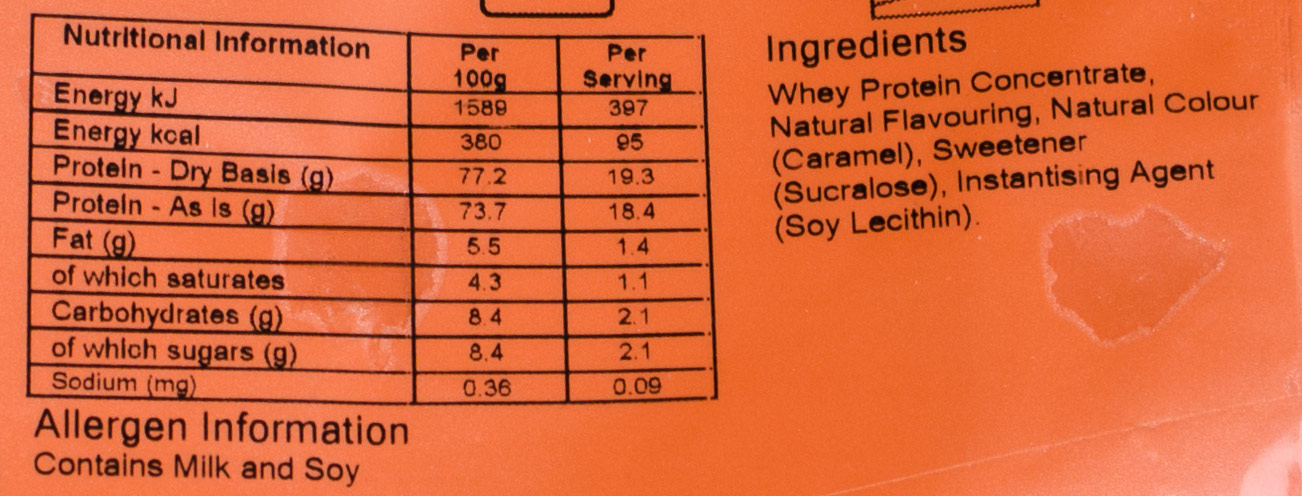This horizontally cropped color photograph depicts the nutritional label of a packaged food product. The image prominently features a contrasting color scheme of orange, black, and bright white, making the information easily readable. On the left-hand side of the label, a grid outlines the nutritional information, with two columns labeled "per 100 grams" and "per serving," detailing the values for various nutritional elements such as fat, carbohydrates, and sodium.

Beneath the nutritional grid, allergen information is clearly stated, indicating that the product contains milk and soy. On the right section of the label, the ingredients are listed in detail, which include whey protein concentrate, natural flavoring, natural color (caramel), sweetener (sucralose), instantizing agent, and soy lecithin. The background of the label is an orange hue, slightly marred by light white watermarks or stains, adding texture to the overall appearance of the package.